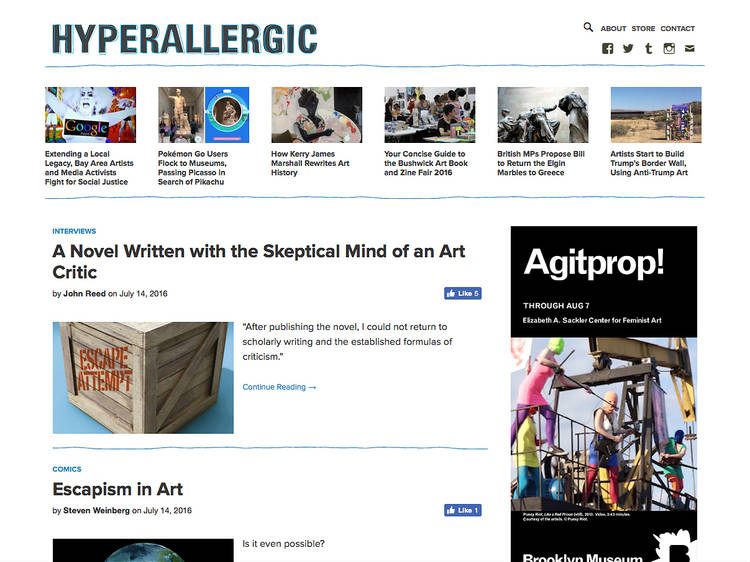**Caption:**

The webpage features a prominent title, "Hyperallergic," styled with black text outlined in blue against a clean white background. In the top-right corner, navigation options include "About," "Store," "Contacts," and social media buttons for Facebook, Twitter, Telegram, Instagram, and Email, followed by a search button.

Below the header, articles are displayed in a horizontal row from left to right. The first article, "Extending a Local Legacy: Bay Area Artists and Media Activists Fight for Social Justice," highlights social justice efforts in the Bay Area. The second article, "Pokémon Go Users Flock to Museum, Passing Picasso in Search of Pikachu," explores the intersection of the tech phenomenon with traditional art spaces. A third article, "How Kerry James Marshall Rewrites Art History," delves into the influential artist's impact. The fourth article, "Your Concise Guide to the Bushwick Artwork Book," offers insights into Bushwick's thriving art scene.

Further down, a list of articles begins with an interview titled "A Novel Writing with the Skeptical Mind of an Art Critic by John Rigg," published on July 14, 2016. This piece discusses the author's shift from scholarly writing to novel writing. Adjacent to this text is an image of a wooden box stamped with "Escape Attempt" in red. The brown box is paired with a blue-patterned design labeled "Escapism in Art by Stephen Weinberg," dated July 14, 2016, posing the question, "Is it even possible?"

On the right side of the page, an advertisement announces "Arcade Prop through August 17" at the Elizabeth A. Sackler Center for Feminist Art.